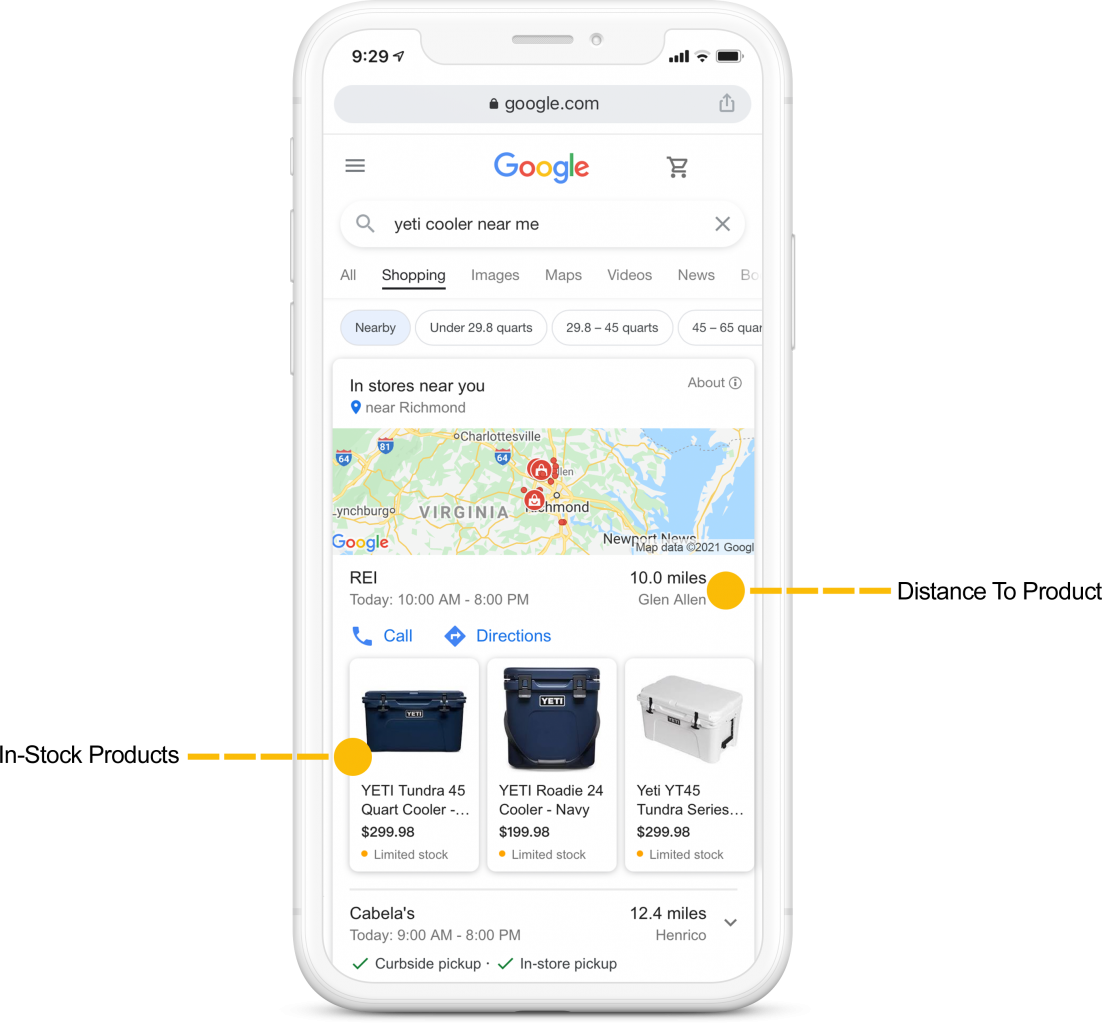In the screenshot, we observe a detailed Google search page at 9:29, presumably either in the morning or evening, indicated by the standard signal, Wi-Fi, and battery icons at the top of the screen. The Google search bar is prominently displayed, featuring the familiar magnifying glass icon on the left side and an 'X' for clearing the search query on the right. The search input currently reads "Yeti cooler near me." Adjacent to the search bar is the Google logo and a shopping cart icon.

Below the search bar, several tab categories are available for refining the search: "All", "Shopping", "Images", "Maps", "Videos", and "News." The user has likely selected one of these tabs, leading to search results categorized under various sections.

In the main results area, there are listings for Yeti coolers by quart size: 2.9.8 quarts, 2.9.8 to 45 quarts, and 45 to 65 quarts. Following this, a section titled "In-stores near you" shows proximity-based results for Richmond, Virginia, along with a clickable map.

The first store listed is REI, located approximately 10 miles away in Glen Allen, open from 10 AM to 8 PM today. This listing includes hot buttons for calling the store and retrieving directions. Furthermore, the store provides a list of in-stock products, spotlighting the Yeti Tundra 45-quart cooler priced at $299.99, among others.

Below REI, Cabela's is mentioned, situated 12.4 miles away. This store opens at 9 AM and closes at 8 PM, offering options for curbside pickup or in-store pickup.